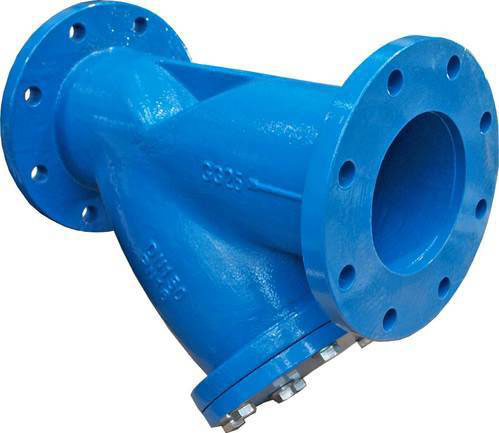The image features a prominent blue, cylindrical steel object set against a completely white background. This heavy, metallic part dominates the center of the image, likely intended to connect hoses or tubes. The object consists of a main cylindrical body with an additional cylindrical piece protruding downward, capped off with a silver end that is secured by screws and likely sealed. Both the main ends of the primary cylinder are open, each surrounded by eight smaller drilled holes for attachment. Visible in the center of the main body are the numbers "3325," indicating possible identification or specification details. The part has areas where it can be bolted or connected, suggesting its use in industrial or home improvement settings.